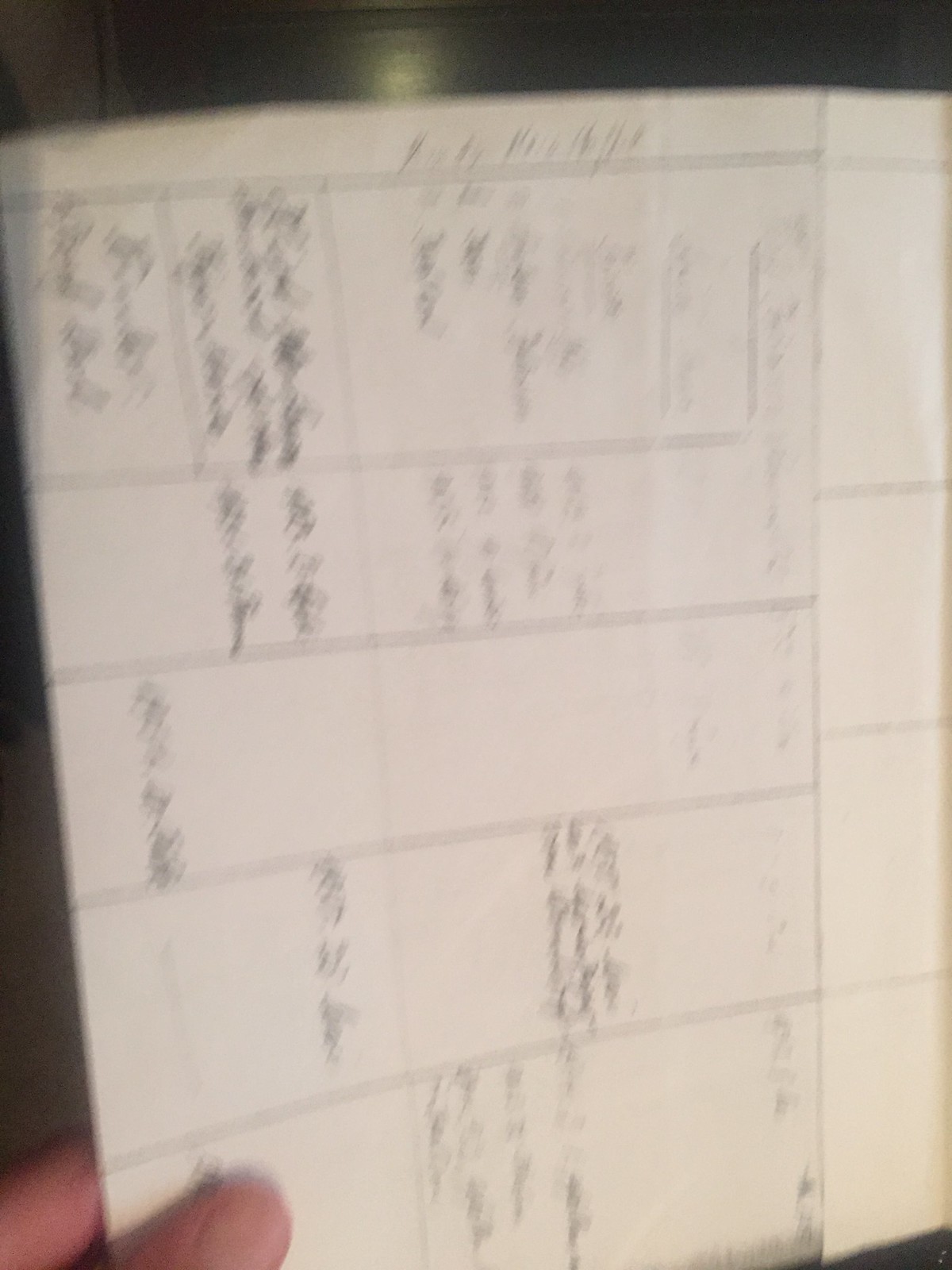The blurred photograph depicts a hand-drawn timetable or calendar on a white sheet of paper, structured into multiple columns and rows by horizontal and vertical lines. Each rectangular section within the grid contains handwriting, likely in black pen or pencil, though the blurriness makes it hard to distinguish. The text appears to be written in cursive and occupies various parts of the rectangles—more writing is noticeable in the leftmost sections, with varying amounts in the middle and right sections. A person's thumb and index finger, possibly belonging to a Caucasian, Hispanic, or Asian individual, can be seen holding the paper in the bottom left corner of the image. The overall image is very blurry, making it difficult to decipher any specific words, but the layout and structure of the timetable are evident.